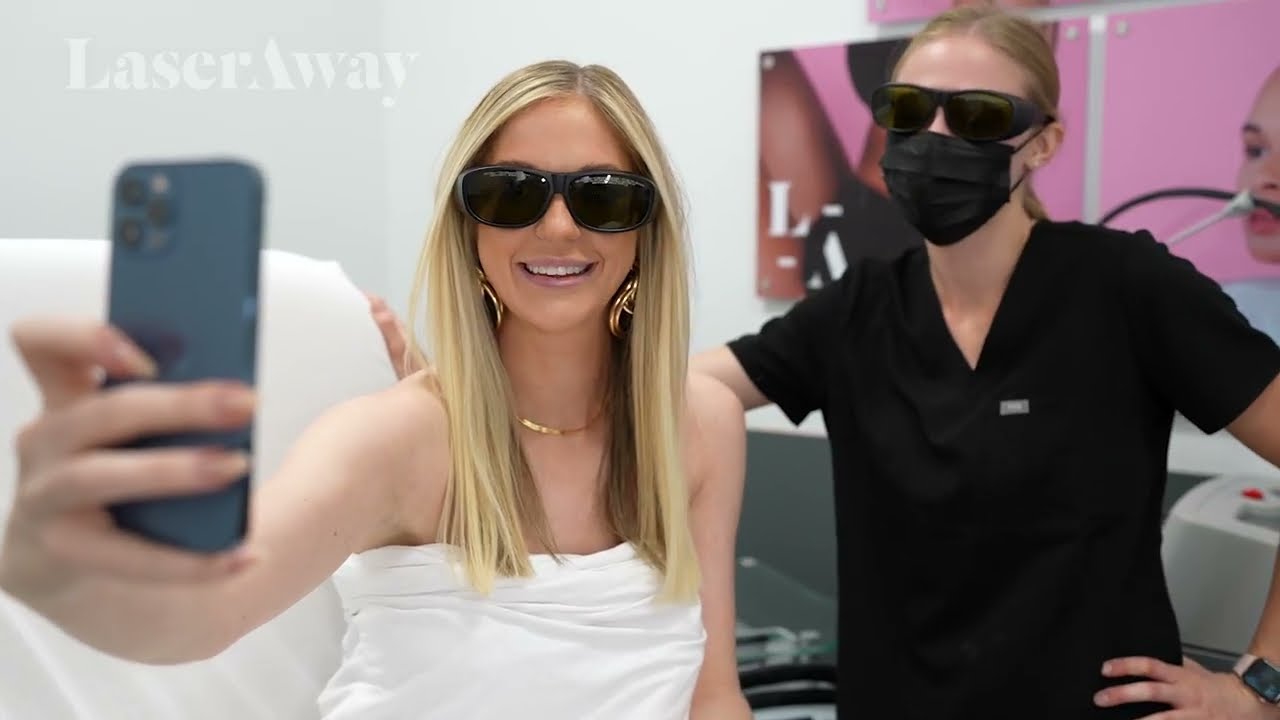The image captures an indoor scene in what appears to be an office specializing in laser hair removal, prominently branded with the name "Laser Away" in white letters in the upper left corner. On the left side of the image is a woman with long blonde hair wearing black sunglasses, gold dangly earrings, a gold necklace, and a white sleeveless top. She is taking a selfie with a gray iPhone, smiling and appearing relaxed, possibly lying in a chair. Standing next to her on the right is a woman who seems to be a technician, identifiable by her black short-sleeved V-neck top, tied-back blonde hair, black sunglasses, and a black surgical mask covering her mouth. The setting suggests a professional environment where cosmetic procedures, like laser hair removal, are performed.